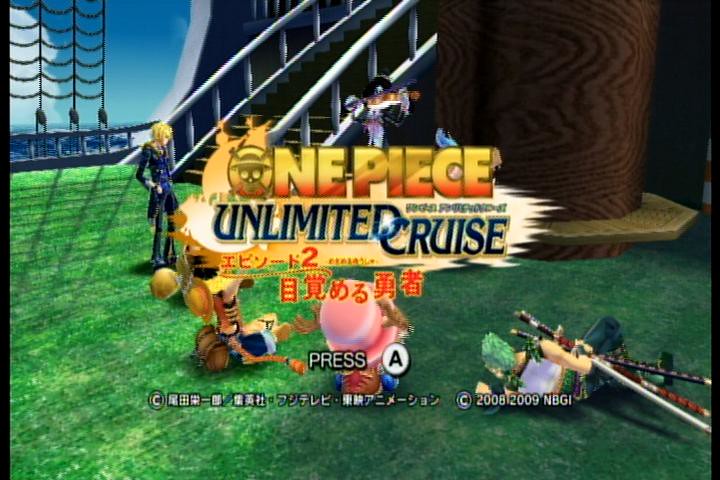**Descriptive Caption:**
A screenshot from the video game "One Piece: Unlimited Cruise" captures a moment from the game's main start menu, as indicated by the on-screen text, "Press A." The image prominently features additional text in Japanese, utilizing Hiragana, Katakana, and Kanji scripts. The game's graphics are notably outdated, characterized by blocky and blurry textures. The scene depicts a grass-covered ship afloat on the sea, integrating elements of natural and nautical themes. Among the five visible characters, one is prone on the deck with multiple swords, while another character resembles a pirate. Due to the general blurriness of the image, it is challenging to discern specific details and features of the characters.